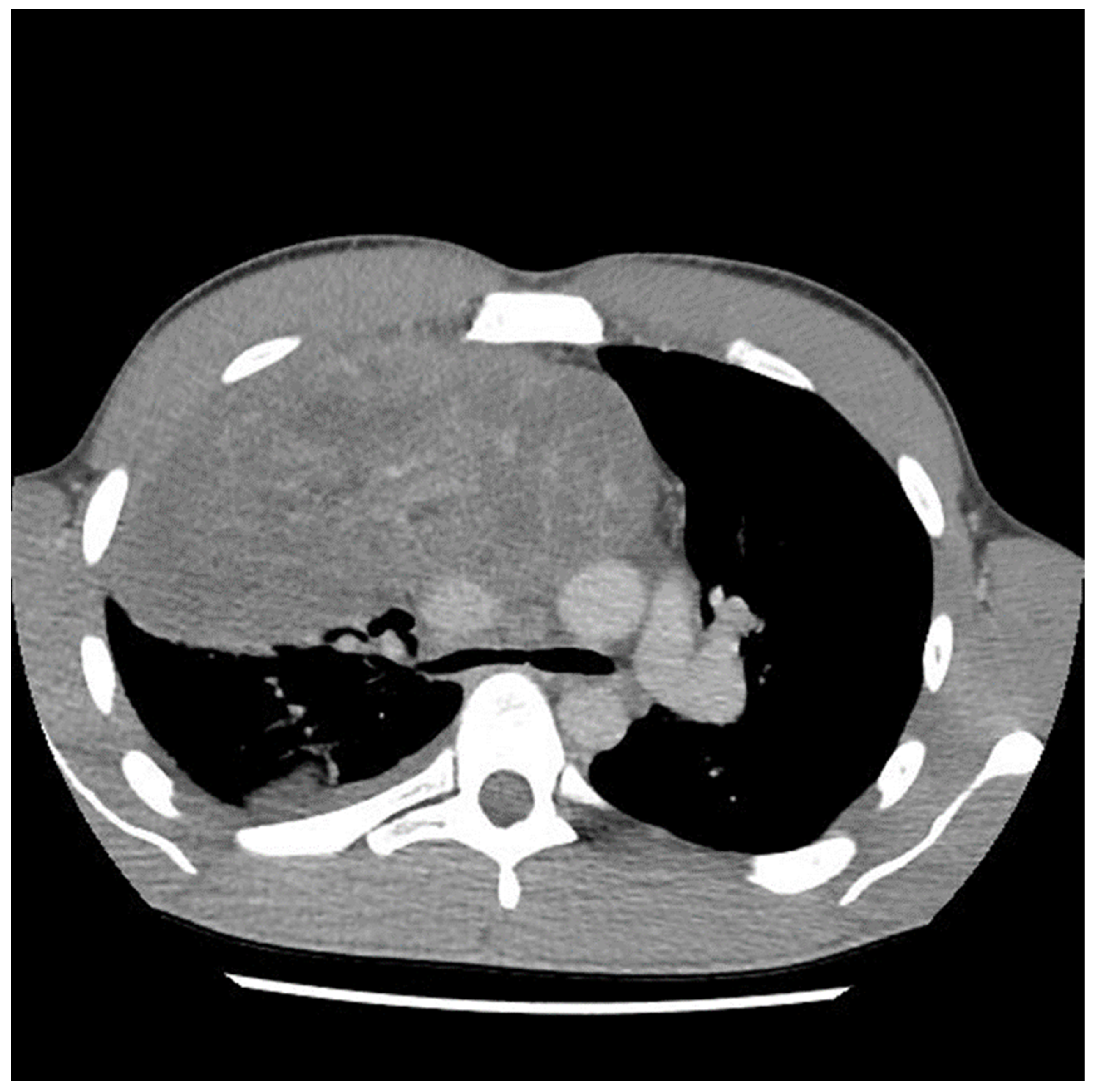The image appears to be a black and white X-ray or MRI scan showcasing a detailed view from a combination of angles, primarily from the top and a semi-side perspective, focusing on the abdominal region. At the bottom of the image, one can distinctly see the patient's hip bones and tailbone. Dominating the center of the scan is a large, elliptical mass with intricate features. This mass appears to be developing, with visible hand-like structures, including fingers, indicating growth. The mass is outlined with scattered white spots or lines, giving it a textured appearance against the predominantly black background. Additionally, there is a straight white line running across the lower portion of the image, providing a stark contrast to the overall scene. Within the central mass, there seems to be a smaller, gray object with a configuration resembling parts of a skull, complete with lighter patches on its sides, enhancing the complexity of the image. The entire presentation gives an impression of an abstract yet medically intricate visual.